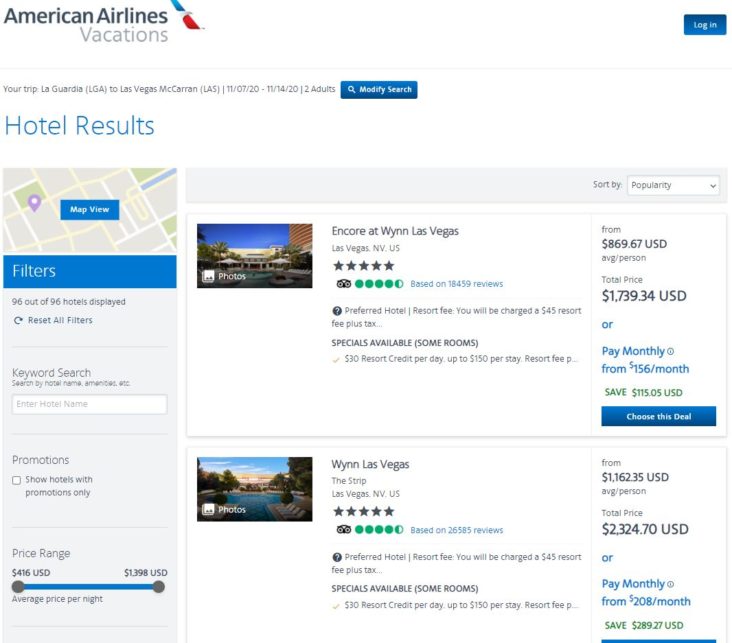In this screenshot from the American Airlines Vacations website, we see the results of a hotel search for a trip from LaGuardia Airport to Las Vegas McCarran Airport, scheduled from November 7, 2020, to November 14, 2020, for two adults. At the top of the page, right under the American Airlines Vacations logo, the details of the trip are displayed. The search results showcase two large, prominent hotel options.

The first hotel listed is the Encore at Wynn Las Vegas, a five-star hotel, with a total price of $1,739.34 for two people for the entire stay. The second option is the Wynn Las Vegas, located on the Strip, also a five-star hotel but with a higher total cost of $2,324.70.

On the left side of the screen, there is a filter section that provides additional search options, including promotions and price range adjustments, allowing users to further customize their hotel search results.